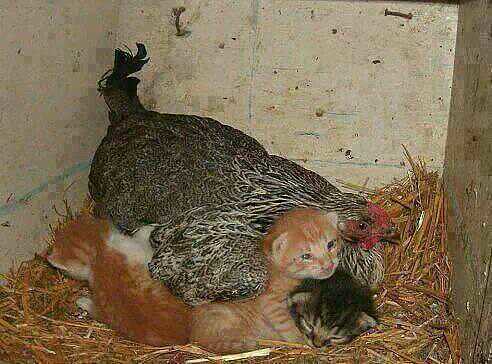An enchanting photograph captures a nurturing scene of a large gray hen huddled over three kittens inside a rustic, white-painted wooden enclosure with visible wear and markings. The hay and grass beneath them provide warmth as the hen, with her red face and black-and-white feathers, appears to be adopting the kittens. One orange-and-beige kitten looks directly at the viewer, while another orange kitten buries its face into the hay. A third kitten, with dark gray and tan fur, completes the trio. The hen lovingly covers the kittens, suggesting a mutual acceptance as if the kittens believe her to be their mother. The enclosure seems cozy, with a light blue line running through its backdrop, emphasizing the close-knit, heartwarming scene of interspecies bonding.